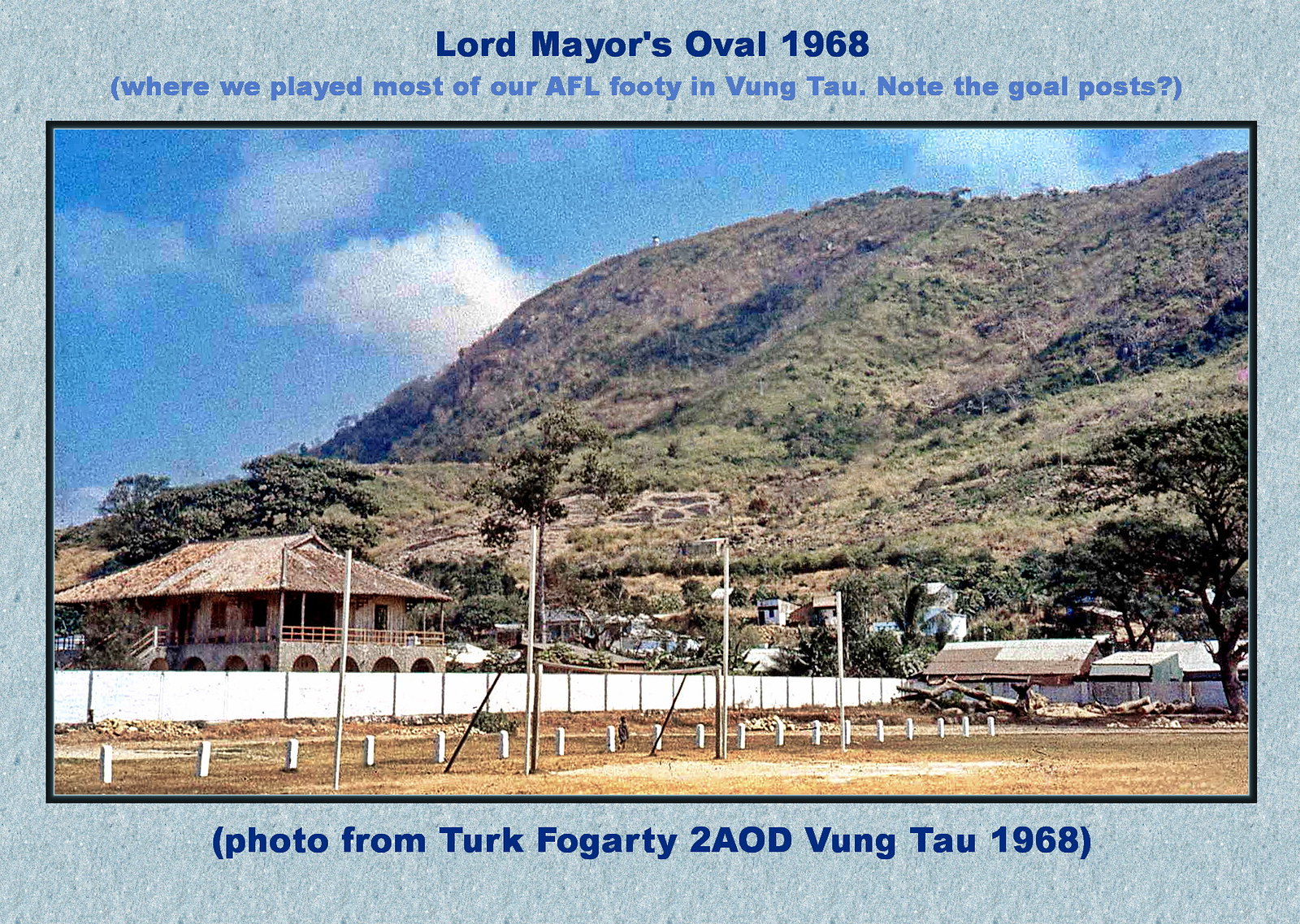**Lord Mayor's Oval, 1968**

This nostalgic image, captioned "Lord Mayor's Oval, 1968" with a note, "where we played most of our AFL footy in Vung Tau," captures a moment steeped in history and natural beauty. The foreground prominently features a pair of wooden goalposts on a field, emphasizing its use for AFL footy games. To the left of the goalpost, a towering, hilly mountain dominates the background, covered in lush green foliage. Below the mountain, to the left side of the image, a brown, two-story building with a triangular roof stands out. This building features arc-shaped doors on the ground level and a porch on the second level, hinting at its old, rustic charm. Adjacent to this building is a white fence, behind which another house and a tall tree can be seen, further enhancing the picturesque quality of the scene.

Adding to the postcard-like quality of the image, the sky above the mountain is a brilliant blue with scattered white clouds, creating a serene and timeless backdrop. The elements combined, from the wooden goalposts to the historical note, weave a tale of a bygone era of local footy games set against a breathtaking natural landscape.